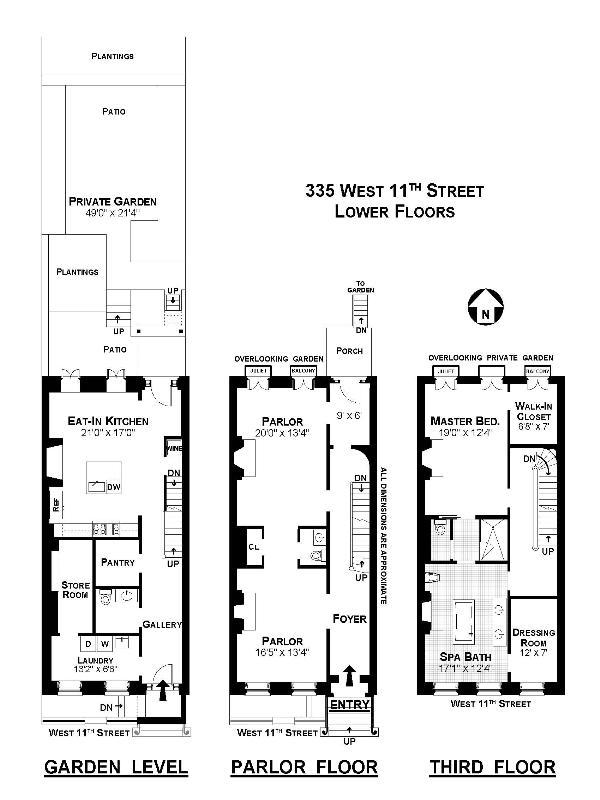Detailed Caption:

This is a detailed, black-and-white digital blueprint of a residential property located at 335 West 11th Street, focusing on the lower floors. 

**Garden Level:** 
- **Top View:** The garden level is illustrated, showcasing various components. 
- **Exterior Areas:**
  - **Plantings:** Areas designated for garden greenery.
  - **Patio:** An outdoor sitting area adjacent to the garden.
  - **Private Garden:** A secluded garden space towards the rear.
  - **Additional Plantings and Patio:** More garden spaces and an additional patio further back.
- **Interior Areas:**
  - **Eating Kitchen:** A kitchen designed for dining.
  - **Gallery:** A hallway leading to other rooms.
  - **Pantry, Storeroom, and Laundry:** Utility spaces for storage and laundry purposes.

**Parlor Floor:**
- This section lies centrally on the map.
- **Parlor Rooms:** Two large parlor rooms indicated at the top.
- **Foyer:** An entry area leading into the residence.
- **Porch:** An outdoor extension accessible from this level.

**Third Floor:**
- **Master Suite:** Contains a master bedroom with an adjoining walk-in closet.
- **Luxury Amenities:** Includes a spa bath and a dressing room.
- **View:** Overlooks the private garden situated on the garden level.
- **Directional Cue:** The top of the blueprint features a compass indicator (circle with an arrow) pointing North (N).

Overall, this map serves as a comprehensive layout of the described residence's lower floors, meticulously detailing both the interior and exterior architecture.